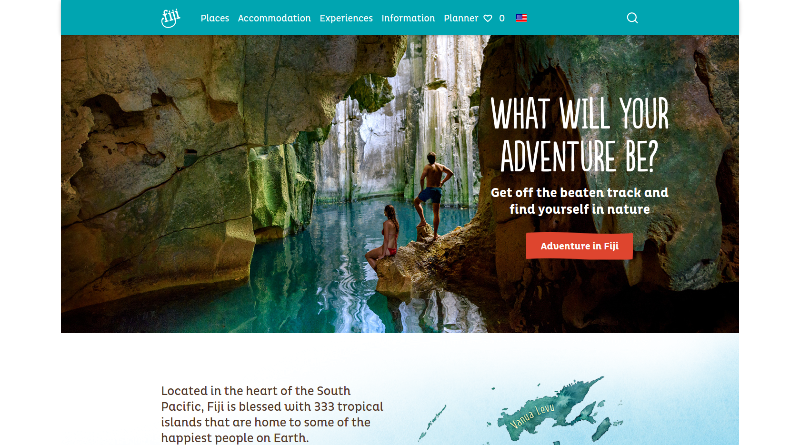The rectangular image, oriented with its longer side running horizontally, features a distinct turquoise bluish-green banner across the top. This banner contains skewed white text reading "Fit" encircled, followed by "places," "accommodation," "experiences," "information," and "planner." It also includes a heart, a flag, and a search icon on the right.

Beneath the banner, the text "What will your adventure be? Get off the beaten track and find yourself in nature." is prominently displayed in white. Below this, a red box with white text declares "Adventure in Fiji."

The main image showcases a serene scene of a woman seated on a rock at the edge of an indoor lake, surrounded by caves and rocky formations. A man stands just behind her, adding to the sense of shared exploration.

Another banner below this scene reads: "Located in the heart of the South Pacific, Fiji is blessed with 333 tropical islands that are home to some of the happiest people on Earth." To the right, a depiction of some of Fiji's islands appears, set against a light blue background, emphasizing their oceanic setting.